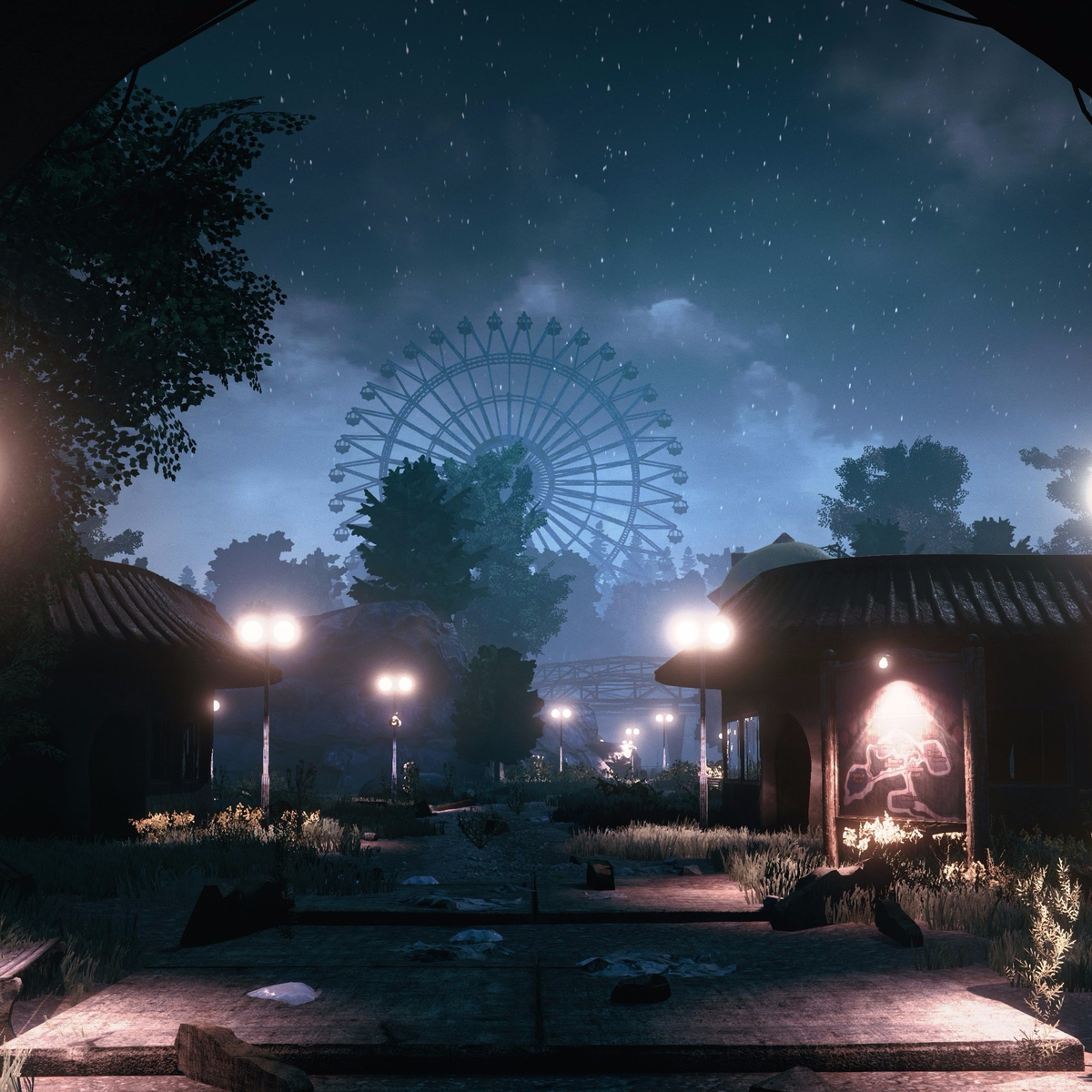This is a detailed nighttime illustration of an abandoned amusement park under a star-studded sky. The dark blue, hazy sky is dotted with numerous stars and delicate clouds, creating a serene yet eerie backdrop. At the center of this scene, the tall silhouette of a Ferris wheel contrasts starkly against the sky. The Ferris wheel, light blue in color, looms in the extreme background, lending a ghostly charm to the scene.

In the foreground, a central wooden walkway, strewn with bits of litter like white plastic bags, extends through the deserted fairground. Flanking this path are patches of overgrown grass and brush, enhancing the abandoned atmosphere. The walkway is lined with street lamps featuring twin globes of light that cast a soft glow on the path, creating guiding beacons through the otherwise barren landscape.

To either side of the walkway stand dark, shadowed buildings, each with flat, slanted roofs and arched doors. These structures, though dimmed inside, have their exterior lights switched on, casting a low light on their façades. One of the buildings in the foreground holds a map of the park, hinting at its past vibrancy. Sparse trees and decorative bushes border these buildings, their silhouettes adding depth to the eerie scene. Overall, the image captures the forlorn beauty of an abandoned amusement park beneath a mesmerizing, starry night sky.